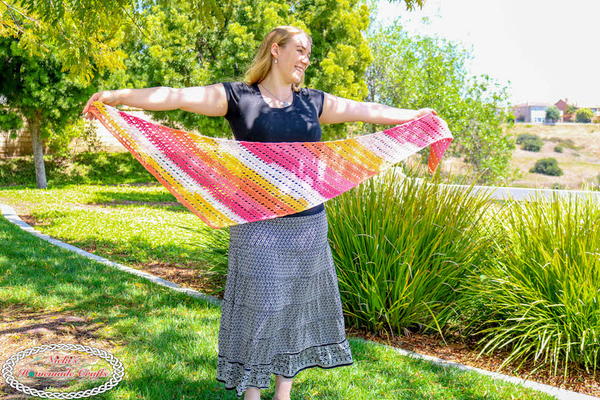This image captures a young blonde woman standing in a park-like setting. She is wearing a navy blue t-shirt and a light blue, almost gray, loosely knit skirt that falls to her ankles. Her attire is accessorized with small earrings. She has outstretched arms, holding a vibrant striped shawl or scarf featuring colors such as pink, orange, yellow, and white arranged in intricate, alternating patterns. She stands on a well-kept grassy area, with rich green bushes and a couple of robust trees behind her. In the mid-ground, there's a path or stepping stones leading towards more bushes and a little building that’s slightly visible in the background. There is also a watermark or logo in the bottom left corner with a Celtic knot border, difficult to read but possibly indicating "Nikki's something," hinting that this image could be part of an advertisement for the shawl. The woman, smiling and looking slightly to her left, is captured in a serene moment, showcasing both the shawl and her surroundings.